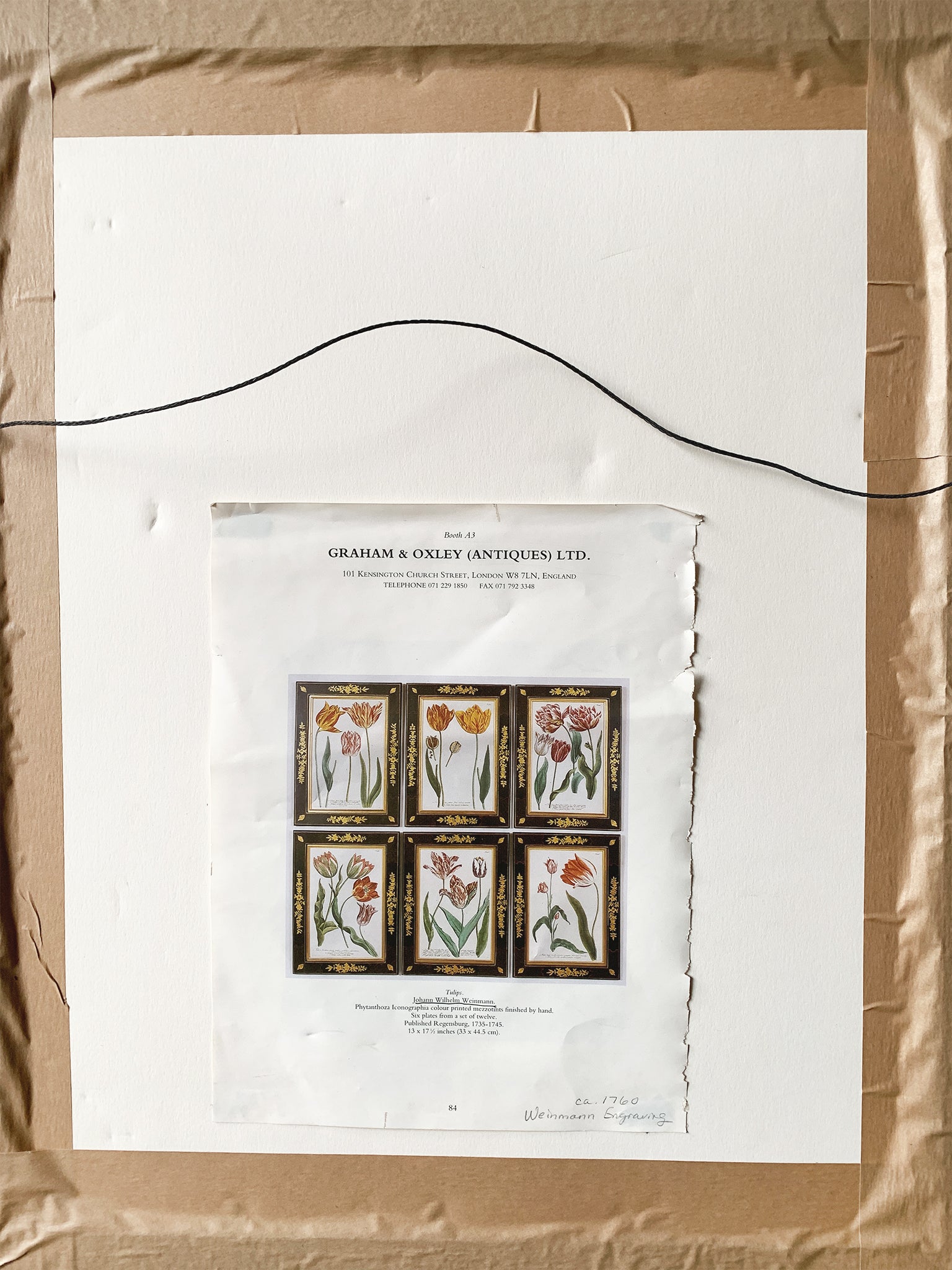The image depicts the back side of a framed piece of artwork. The frame is rectilinear and taped all around with brownish-golden tape, and a black wire strung across about two-thirds up, presumably for hanging. The back is covered with a tight brown paper or fabric. Centered in the back of the frame, a large white poster board or piece of paper is glued, displaying a grid of six images in a three-by-two arrangement. Each image features different flower illustrations bordered by black frames adorned with gold decor at the corners and sides. The text at the top of this paper reads, "Booth A3, Graham and Oxley Antiques Ltd," along with their address, phone number, and fax. There's a description at the very bottom in small, difficult-to-decipher text, with a handwritten note on the bottom right stating, "Circa 1760 Wineman Engraving." The images show various floral compositions, including orange and red flowers, tulips, and possibly a gigantic red flower among others, hinting that the actual canvas could be one of these designs.